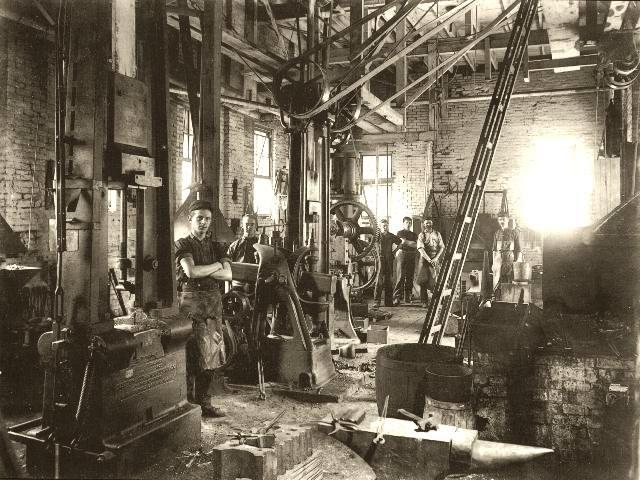This black-and-white image depicts an industrial scene from the early 20th century, capturing a group of approximately half a dozen men hard at work inside a high-ceilinged factory with brick walls. The men are dressed in rolled-up, long-sleeve button-down shirts and long aprons, indicating their roles likely as machinists or workers engaging with the heavy machinery that fills the space. They wear caps and austere expressions as they look toward the camera, and various tools, belts, pulleys, and machines surround them, whose exact purposes are not entirely clear. Prominently featured is a large ladder extending from the floor to the wood-planked ceiling and several barrels scattered throughout the room. The overall impression is of a diligent workforce operating in a robust, mechanical environment, frozen in a moment of determined activity.